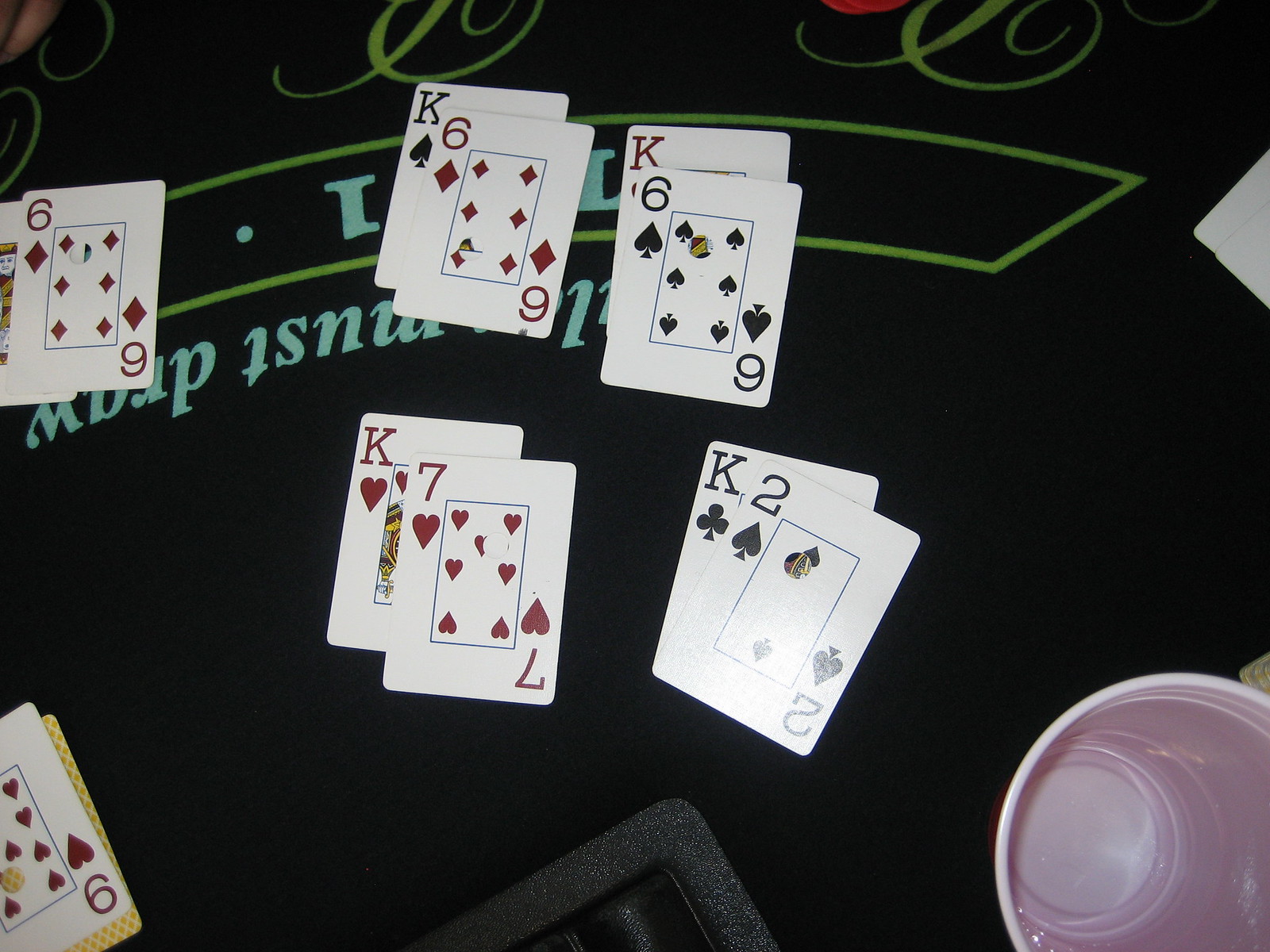In an indoor setting, centered around a green felt poker table, a detailed scene unfolds. The table displays a variety of playing cards laid out in a specific order. From left to right, the visible cards include a six of diamonds and partially hidden beneath it, a king of spades. Following this, we see a standalone king card (king of hearts), a six of spades underneath those cards, and further along the table, a two of spades paired with a king of clubs. Close to these, there is a seven of hearts positioned next to a king of hearts, and finally, a nine of hearts partially obscured by another card. At the bottom center of the photo, there is a small chip tray, while the lower right corner features an empty red solo cup. The image captures the essence of a tense poker game in progress.